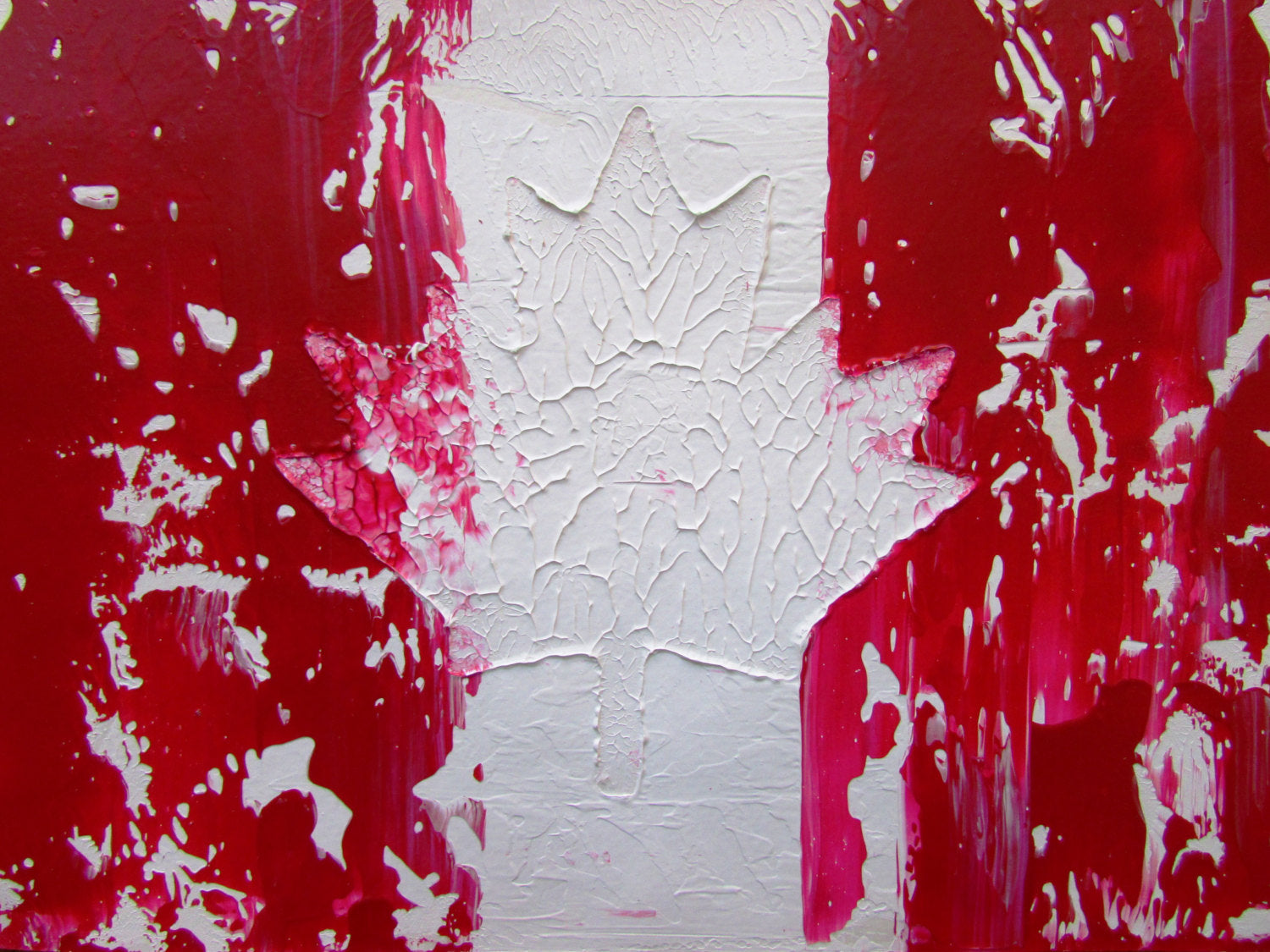This image, in landscape layout, features a central white section with a textured, intricately drawn leaf, possibly a Canadian maple leaf, etched in fine detail with thin white paint strokes, revealing delicate roots within. Flanking this central white area are vertical bands on the left and right, covered in a red material—likely plastic—with splatters of white paint. The red sections have white splotches breaking through, suggesting an intentional but somewhat messy overlay. The entire composition creates a stark contrast between the textured white center and the vibrant red sides, giving the appearance of a rectangular painting devoid of other colors, text, or borders.